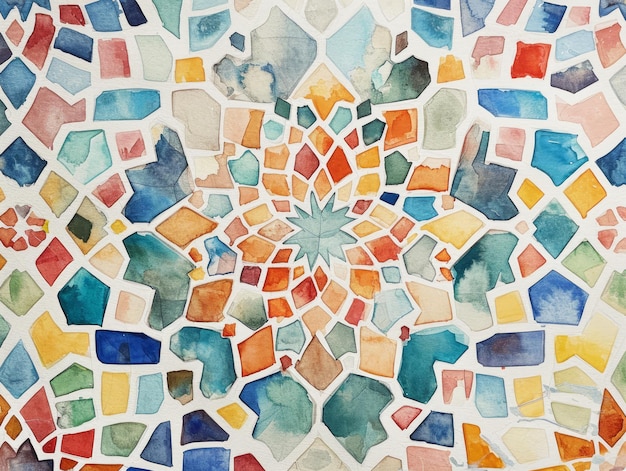This abstract watercolor painting, reminiscent of a mosaic, captures a vibrant and intricate array of colors and shapes. Dominated by an expansive design that would ideally hang in a living room, the artwork features a central motif—a starburst or flower-like shape—in shades of blue, teal, and green. Radiating outward, irregularly shaped "tiles" of peach, red, yellow, green, gray, and burnt orange spread across the canvas, their edges defined by bands of white, mimicking grout in a traditional mosaic. The background remains predominantly white, enhancing the mosaic effect created by the fragmented patches of color. This elaborate watercolor composition showcases a harmonious blend of hues and forms, extending seamlessly across the entire space without any framing, creating a stunning visual tapestry.